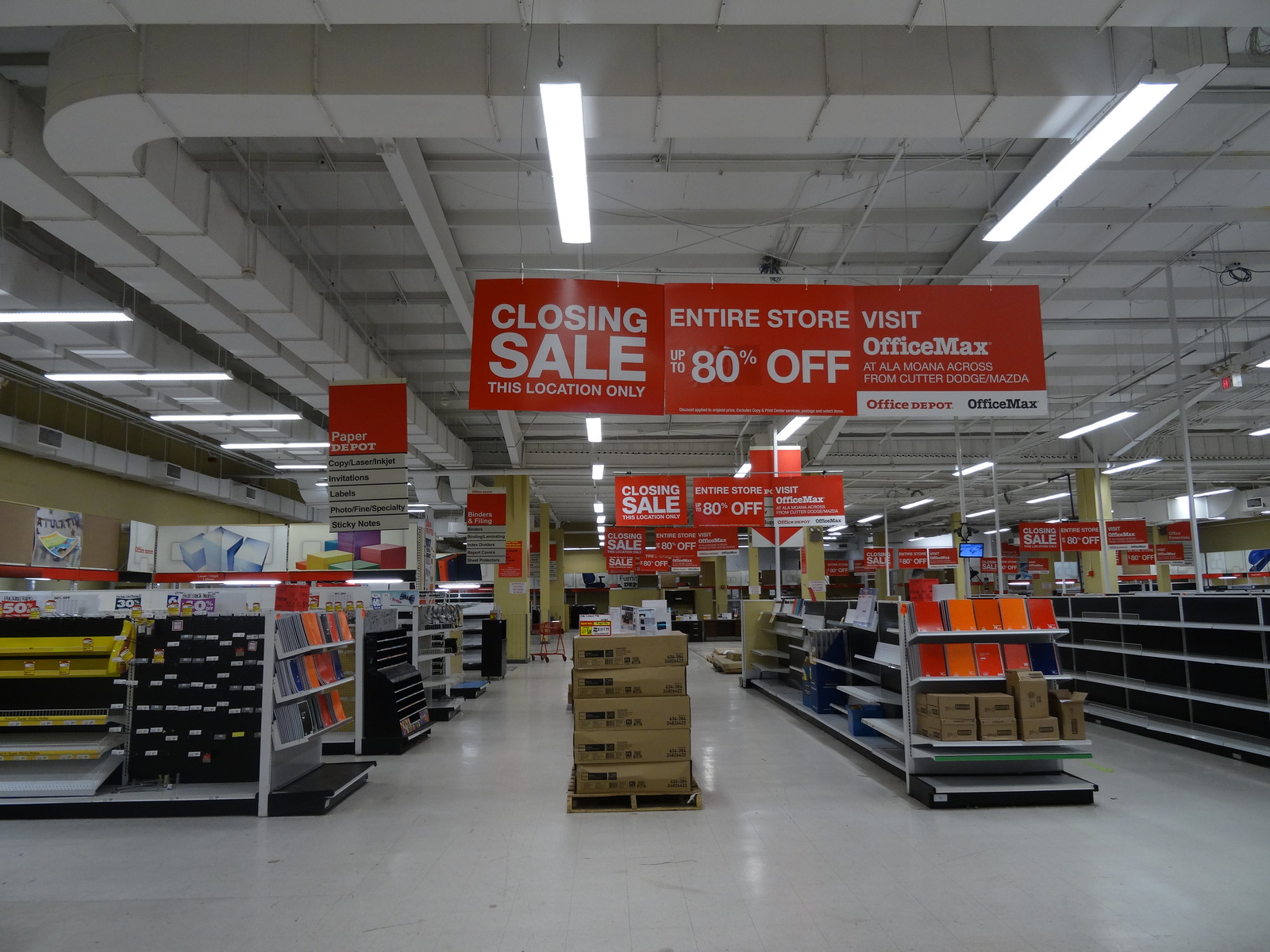The photograph captures the interior of a large department store, specifically an OfficeMax, illuminated entirely by fluorescent lights. Dominating the scene is a prominent red sign that reads, "Closing Sale: Entire Store 80% Off." The store is well-organized with visible aisles stocked with various office supplies, including notebooks, pens, and folders. The atmosphere feels somewhat isolated, as no people are noticeably present, though a closer inspection might reveal a few distant figures. The environment is overwhelmingly artificial, characterized by a pervasive whiteness—from the ceiling and floor to the glaring lights—contrasted sharply by the bold red sale signs. The absence of natural light makes it difficult to ascertain the time of day.